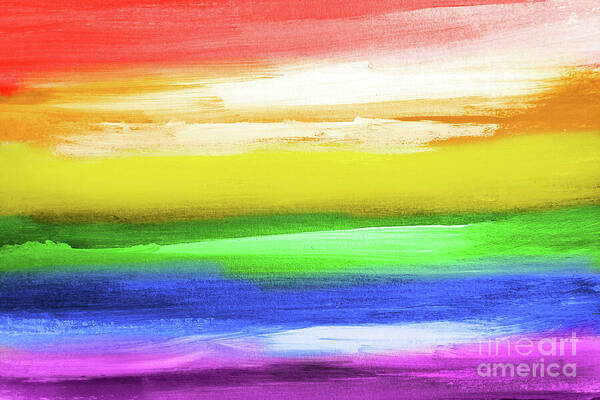This image is a hand-painted depiction of a rainbow, resembling a watercolor artwork. The painting features horizontal brush strokes that transition across the colors of the rainbow. Starting from the bottom, the color bands include purple, dark blue, green, yellow, orange, and red at the top. Within these bands, there are white streaks that add a reflective quality to the image. The brush strokes are evident, enhancing the texture and depth of the piece. In the bottom right corner, there is a semi-transparent watermark that reads "Fine Art America." The overall effect is reminiscent of an ocean scene with waves and hills, interpreted through the various rainbow-colored bands.